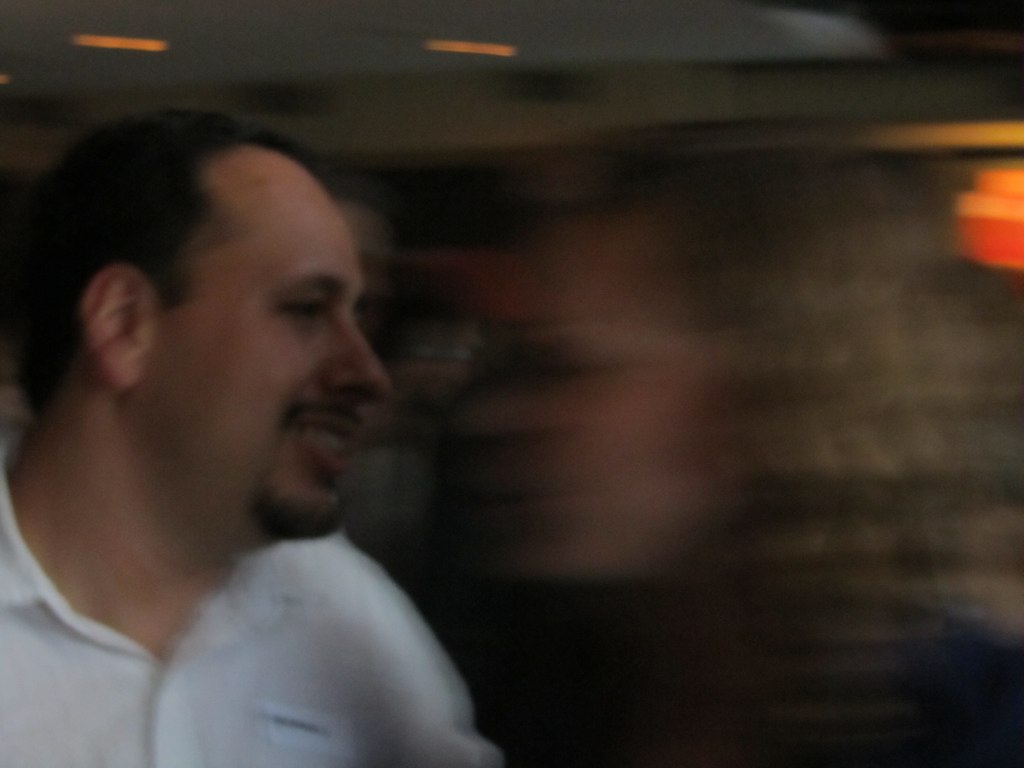The image depicts a man with short, dark hair, a wide forehead, a mustache, and a slight goatee, wearing a white collared polo shirt. He is seen from a side view, looking to his right towards a blurred image of a woman with curly, shoulder-length blonde hair. The woman, clad possibly in a dark or blue-colored top, is less distinct due to the motion-induced blurriness of the photograph, making it difficult to discern the finer details of her face or attire. The scene appears to be either indoors or in a dimly lit area, with various light sources visible. Notably, there are spherical-shaped blurs of light near the top, indicative of ceiling lights, and an orange-red square shape in the background. Additional individuals are faintly visible in the backdrop, further obscured by the image's motion blur, adding to the dynamic, slightly chaotic feel of the photograph.